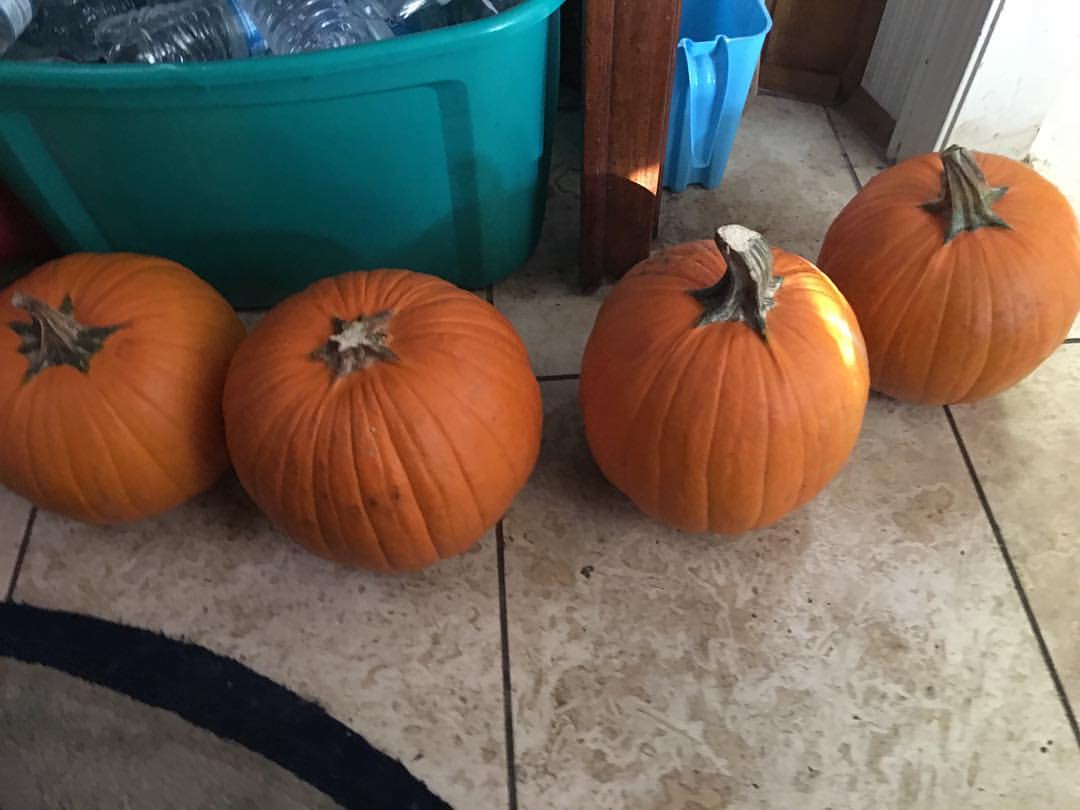This color photograph captures the interior of a space, likely a kitchen, featuring a stone tile floor with a marbled effect. In the foreground, four small, nearly identical pumpkins are arranged in a semi-circle, extending from the left middle portion of the image to the upper right portion. Notably, there is a light spot illuminating the right side of the third pumpkin. Behind the pumpkins, a light blue or greenish-teal Tupperware bin brimming with plastic bottles can be seen, suggesting it might be used for recycling. Additionally, a light blue plastic pitcher is situated on the floor in the top right section of the image. The overall scene has a slightly cluttered appearance and evokes a casual, everyday setting.